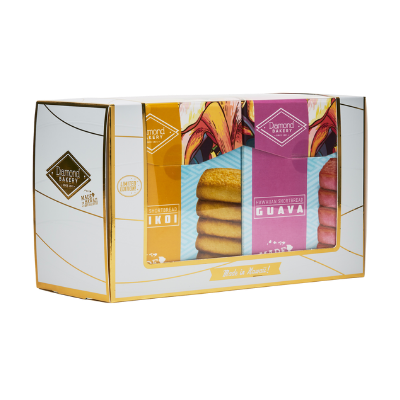This elegant and modern cookie sampler box, likely from Diamond Bakery, boasts a sophisticated design with a white base and tasteful gold accents framing each flap. The box displays images of square cookies, indicating the inclusion of two distinct flavors: a pinkish guava cookie and a yellowish-brown Ikoi cookie. Although the text on the packaging is mostly in a foreign language, the word "guava" is clearly legible, suggesting the exotic nature of these treats. The graphics and contemporary gold and green details on the box further enhance its classy appearance, making it an attractive choice for those seeking a refined snacking experience.